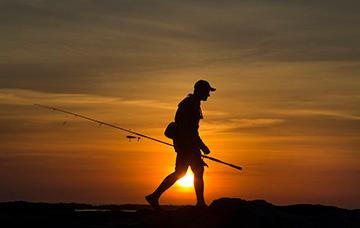A striking photograph captures the silhouette of a tall man walking at sunset under a sky that transitions from dark gray to vibrant orange and yellow. Dominating three-quarters of the image, the skyline is enhanced with dramatic clouds. The setting sun appears through the man’s legs, casting a radiant glow and illuminating the scene. The man, wearing a forward-facing baseball cap and carrying a fishing pole on his shoulder, strides towards the right of the frame. The fishing pole extends diagonally from the bottom right to the top left of the image, with a lure dangling from the back. He carries a backpack, with one heel lifted as he steps forward on the shadowed, flat ground below. The entire scene portrays a tranquil moment, silhouetted against the colorful, descending sun.